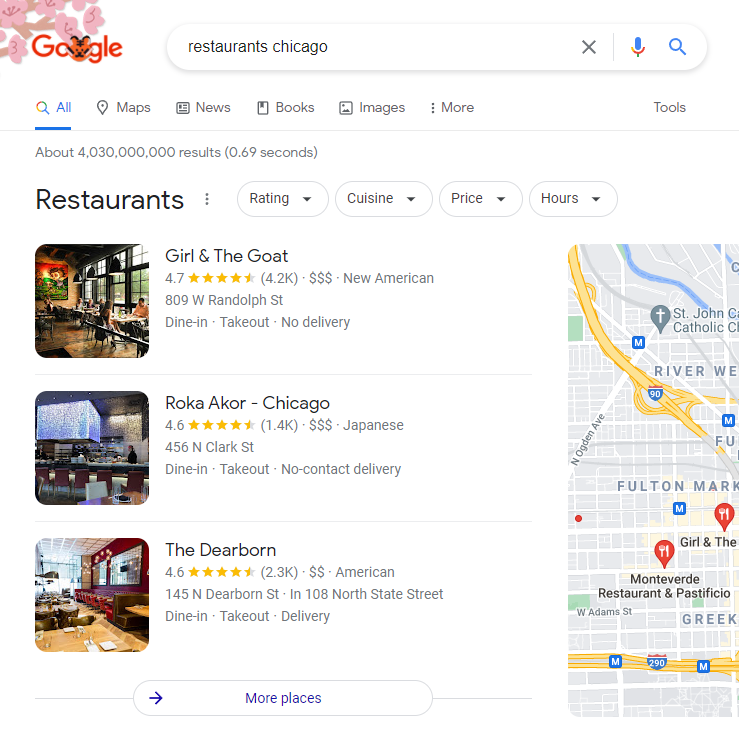A screenshot of a Google search page is displayed, featuring a Google Doodle at the top left corner, depicting a tree adorned with pink flowers and the word "Google" written in red. The search bar contains the query "restaurant Chicago." Just below the search bar, a menu bar includes options labeled "All," "Maps," "News," "Books," "Images," "More," and "Tools." A line spans the width of the page beneath this menu.

The search results indicate approximately 4 billion and 30 million results, retrieved in 0.69 seconds. Following this, filters for refining the search results are available with dropdown menus titled "Ratings," "Cuisine," "Price," and "Hours."

The first search result is highlighted with an image of the restaurant's interior and details about "Girl and the Goat." This establishment boasts 4.7 stars from 4.2k ratings and is categorized under "New American." It is located at 809 West Randolph Street and offers dine-in and take-out services, but no delivery options.

The second result is for "Roca Accor Chicago," rated 4.6 stars based on 1.4k reviews. It is described as a Japanese restaurant with three dollar signs indicating the price range.